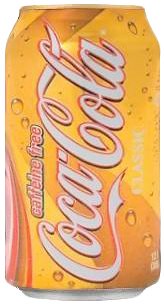This image features a vibrant yellow aluminum can of caffeine-free Coca-Cola. The can's unique design includes numerous transparent bubble illustrations that give it a fizzy, effervescent appearance. The iconic Coca-Cola logo is prominently displayed in elegant cursive, stretching vertically from the bottom to the top of the can. Above the logo, the words "caffeine-free" are presented in small, regular block letters, highlighted in white with a delicate pink hue. An artistic arch composed of pink, yellow, and white lines adorns the left side of the can, extending from the middle to the bottom. The very bottom edge of the can is silver, and the word "classic" is inscribed in white beneath the Coca-Cola logo. This design combines both modern and classic elements, evoking a sense of timeless refreshment.